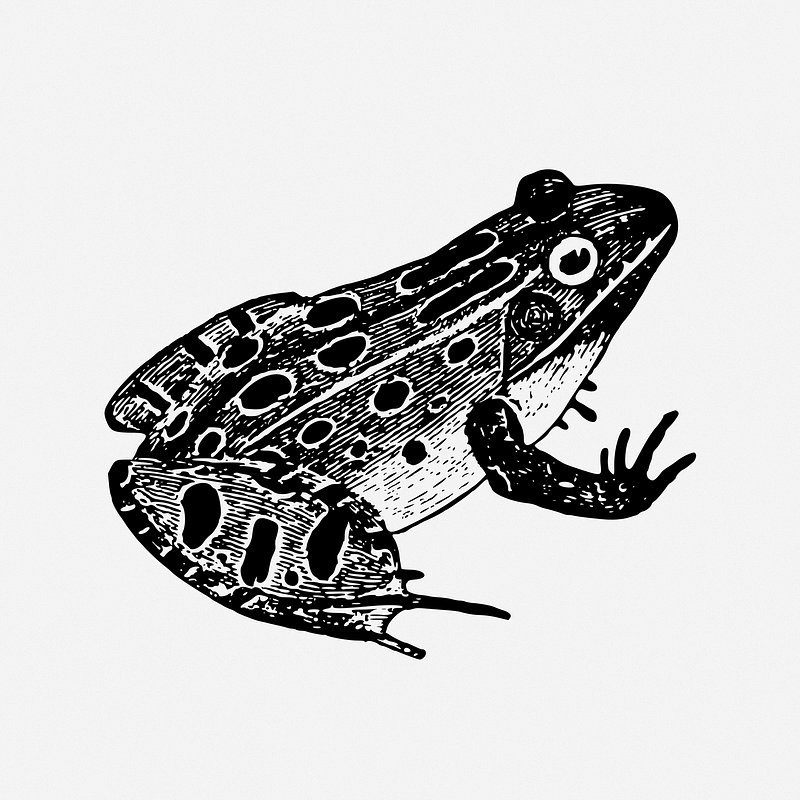The square image features a detailed black and white illustration of a frog, characterized by thick lines and intricate shading. Positioned in profile, the frog's head faces to the right with one large eye, prominent and alert, seemingly on the lookout for flies. Its characteristic large hind legs, essential for hopping, extend towards the left and exhibit rows of black spots along both the legs and the body. The frog’s dark forearms have four fingers each, and its belly contrasts as a lighter, whitish shade, which helps in water protection. The background is a very light grey, almost white, enhancing the frog's distinct markings and the bold lines of this stamp-like illustration. The overall composition highlights the frog's natural features in stark black and white, from its dark face towards the nose to the uniquely striped and spotted pattern on its skin.